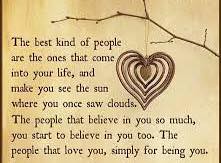The image features a small, simplistic photograph set against a tan, aged-looking background with black text. It is bordered on the left and right sides with a dark brown or black color, matching on both sides. There is no visible border on the top and bottom. A bare tree branch with tiny buds extends from the upper right side of the picture. Hanging from this branch is a heart-shaped ornament, adorned with several concentric rings of smaller hearts within it. The text on the image reads: "The best kind of people are the ones that come into your life and make you see the sun where you once saw clouds. The people that believe in you so much, you start to believe in you too. The people that love you simply for being you." This heartfelt poem is rendered in black text, complementing the nostalgic tone of the beige backdrop, evoking a sense of warmth and simplicity.